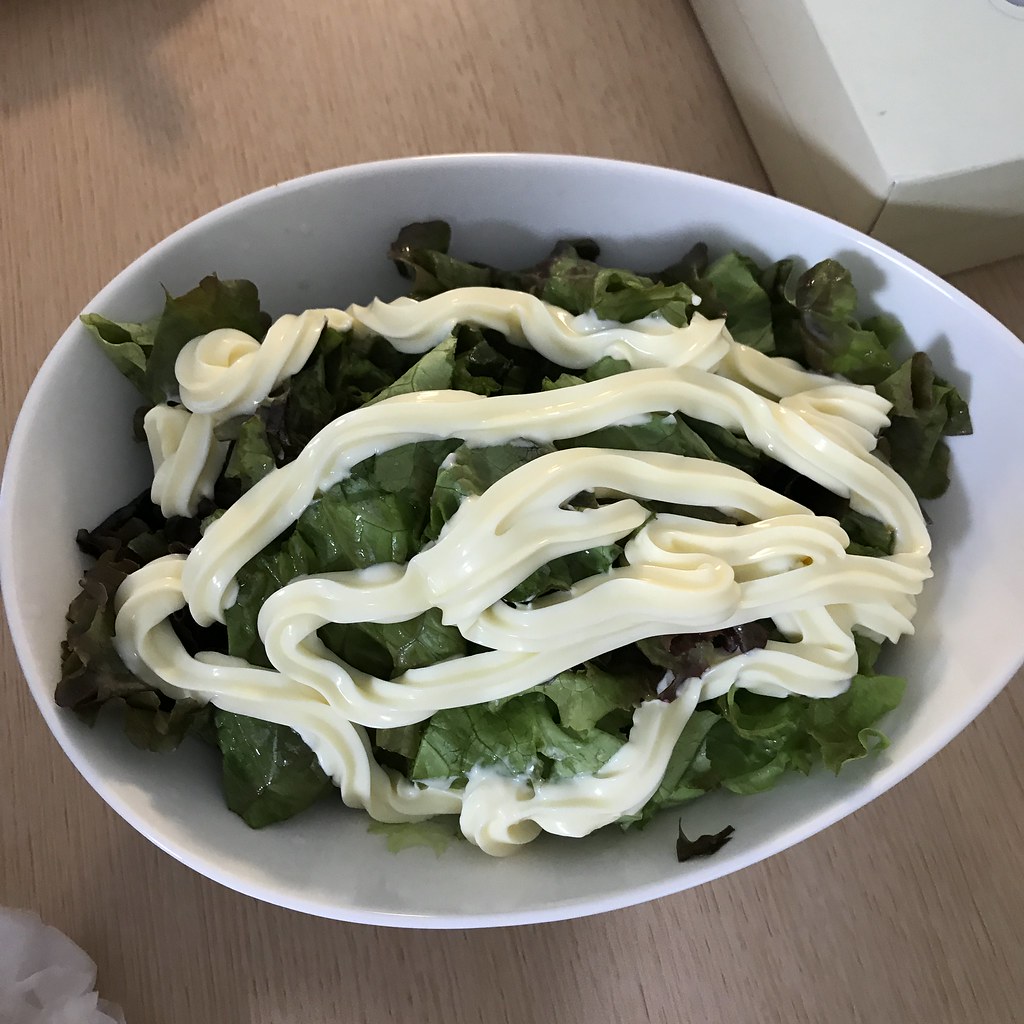This photograph showcases a meal on a light brown wooden surface. Dominating the scene is an oval, egg-shaped, white ceramic bowl positioned centrally, containing a bed of vibrant green romaine lettuce leaves. Generous amounts of chunky, white mayonnaise are squirted across the top of the lettuce. The right edge of the bowl is slightly cut off, but all the food remains visible within the bowl. In the lower left corner, part of a small white box is apparent, while a white object, possibly a flower or napkin, is also visible. Subtle shadows enhance the composition, including one in the top left corner.